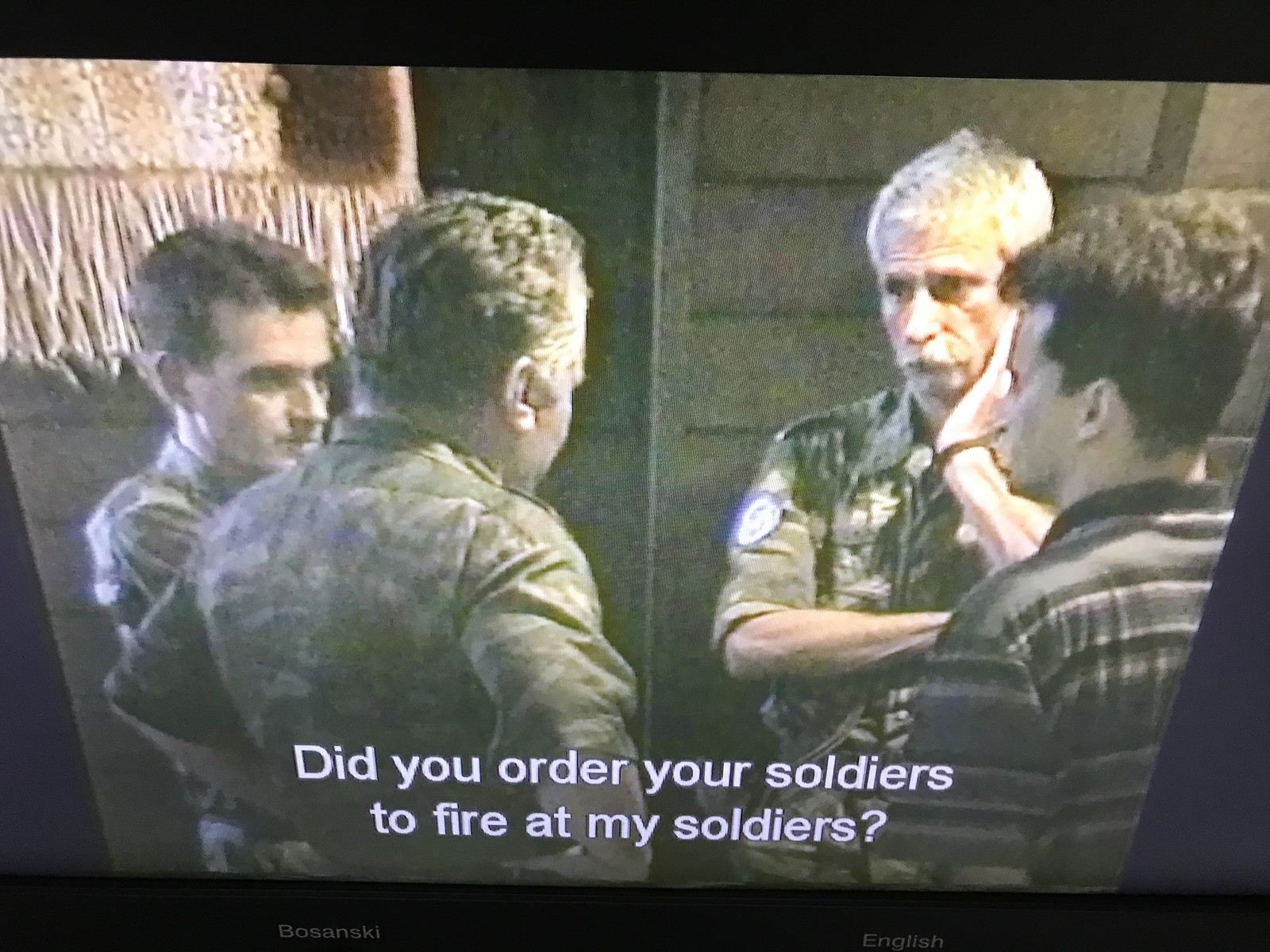The image appears to be a low-resolution photograph of a television screen or movie projection, depicting a nighttime scene with four white men engaged in a serious conversation. Three of the men are dressed in camouflage army uniforms, while the fourth wears a striped polo shirt with black, gray, white, and red horizontal stripes. One of the soldiers is notably older, with gray hair and a gray mustache. The group is huddled together, standing near what looks like a wood-sided cabin with visible side paneling and a window in the background. The white subtitle at the bottom of the screen reads, "Did you order your soldiers to fire at my soldiers?" The man in the bottom left of the screen is speaking to the older man positioned at the top right of the group.